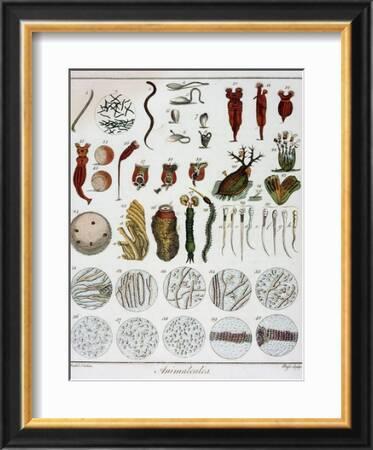The image in question is a framed vintage scientific print, encased in a black frame with a gold border inside and a white mat surrounding the central illustration. The content of the print appears blurry, making the text unreadable, but it features a detailed array of colorful images depicting various scientific subjects. The centerpiece, with a gray background, showcases numerous illustrations, including worm-like structures and possibly parasites, indicating it might be a scientific poster. Additionally, the bottom part of the print contains two rows of five circular images, which seem to be microscopic views, possibly of cells or bacteria. While the exact details are unclear due to the image's blurry nature, the organized layout with numbered labels suggests it is designed for scientific reference.